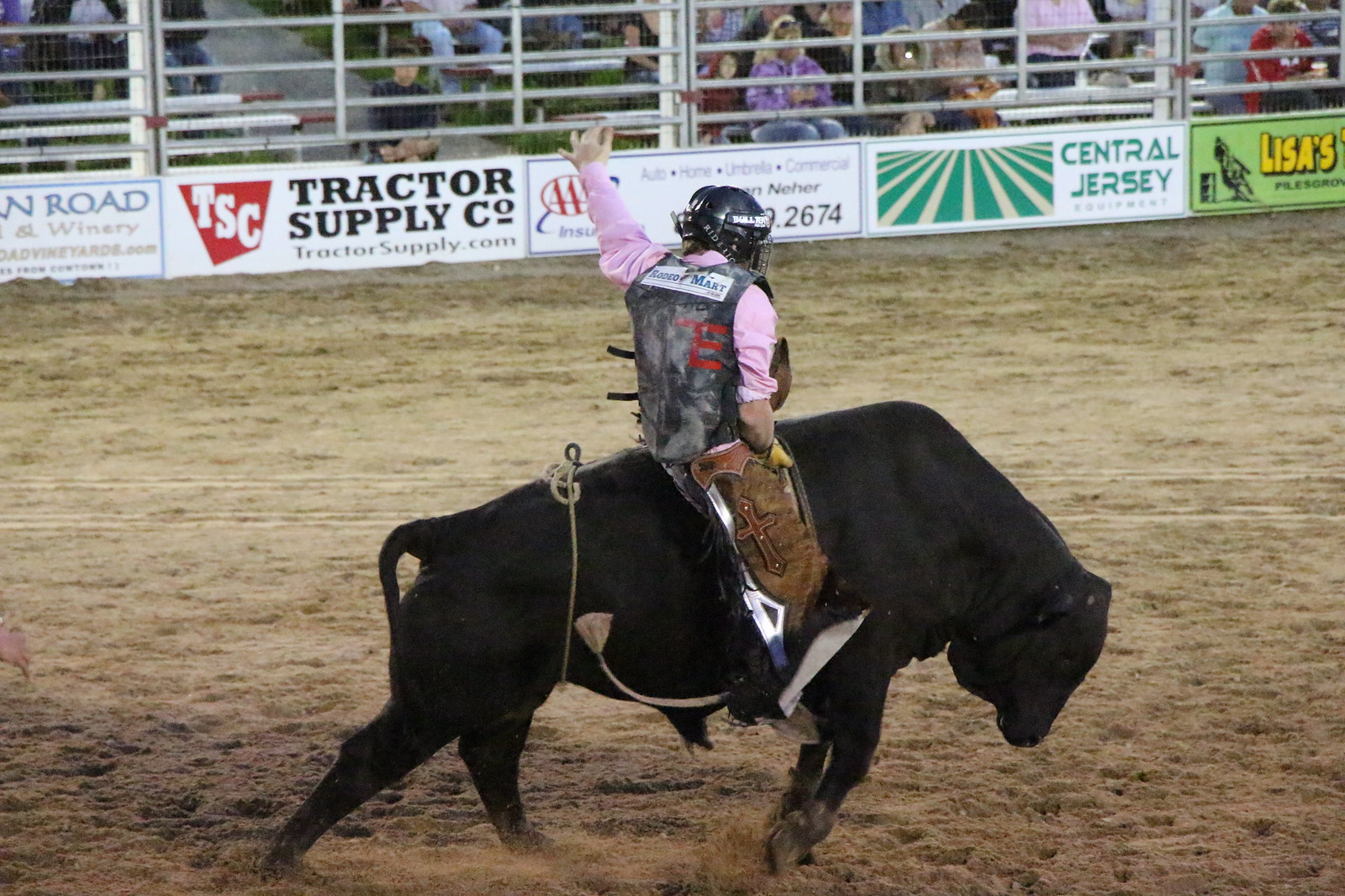This photograph captures an intense moment at an American rodeo, featuring a cowboy skillfully riding a black bull that's mid-buck. The bull's side profile reveals its muscular frame, possibly a Brahma Angus cross, characterized by a slight hump and a dewlap. The rider is clad in a pink shirt, a black safety vest adorned with "Rodeo Martin" and other writings, along with brown leather chaps featuring a cross design and fur trim on one side. His black helmet with a face mask ensures safety, while his right hand grips the bull's rope firmly and his left arm is poised in the air. The backdrop showcases metal fencing to keep the bull contained, with a packed audience watching from the bleachers. The arena's perimeter is lined with a series of advertisements, including names like Tractor Supply Co., Central Jersey, AAA Insurance, a winery, and others, against the backdrop of the arena’s tan dirt floor.